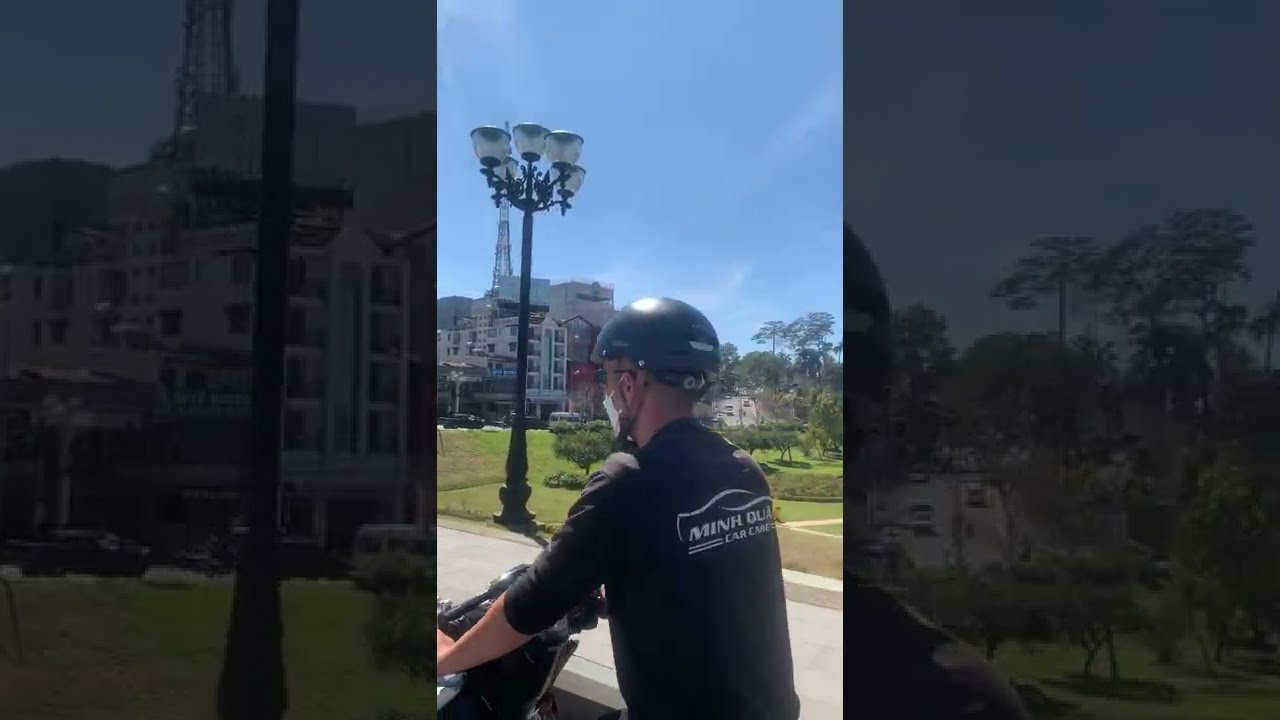A photograph captures a man riding a moped, dressed in a long-sleeve black T-shirt with white lettering on the back that partially reads "M-I-N-H Q-U" followed by "car care." He is wearing a black helmet and a white face mask that covers his mouth. The helmet has a distinctive shine on its top, likely from the sunlight. His shirt sleeves are rolled up to his forearms, and he appears to be wearing glasses as well. The scene is set during the daytime under a clear blue sky, with a few high white clouds visible. To the man's right and on the left side of the photograph, there is a tall black streetlamp with multiple lamps—accounts vary between five and seven. In the background, you can see a sprawling park area with green grass and several trees. Beyond the park, a complex of interconnected buildings, which might be hotels, stands tall. Additionally, a structure resembling a communication tower looms in the distance.